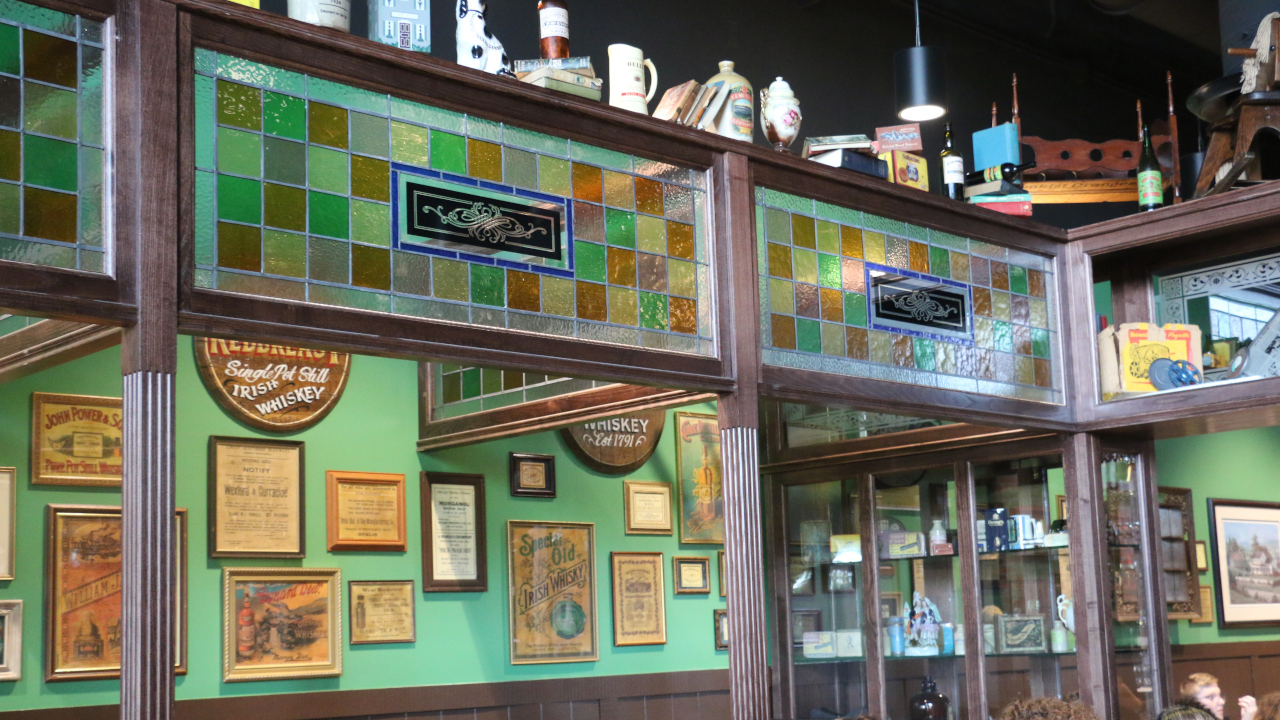The image captures the bustling atmosphere of a cozy restaurant interior, likely a bar, characterized by its distinctive decor and warm inviting ambiance. The background features a green-painted wall adorned with a variety of framed old-school pictures, signs, and documents, creating a nostalgic vibe. Below the frames, a sturdy wood paneling runs horizontally along the wall. At the top of the image, there’s a striking stained glass panel with hues of brown, green, yellow, red, and light blue, adding an artistic touch to the setting. Above this, a shelf houses an eclectic collection of mugs, flasks, pictures, and books. Prominently displayed among the decor is an advertisement for a whiskey brand, with one label reading "Redbreast Single Pot Still Irish Whiskey." On the right side of the image, an all-glass cabinet filled with various items stands out. The warm lighting, provided by hanging lights, complements the cozy environment, with a glimpse of patrons seated at the bottom right corner, further emphasizing the lively and inviting nature of the establishment.